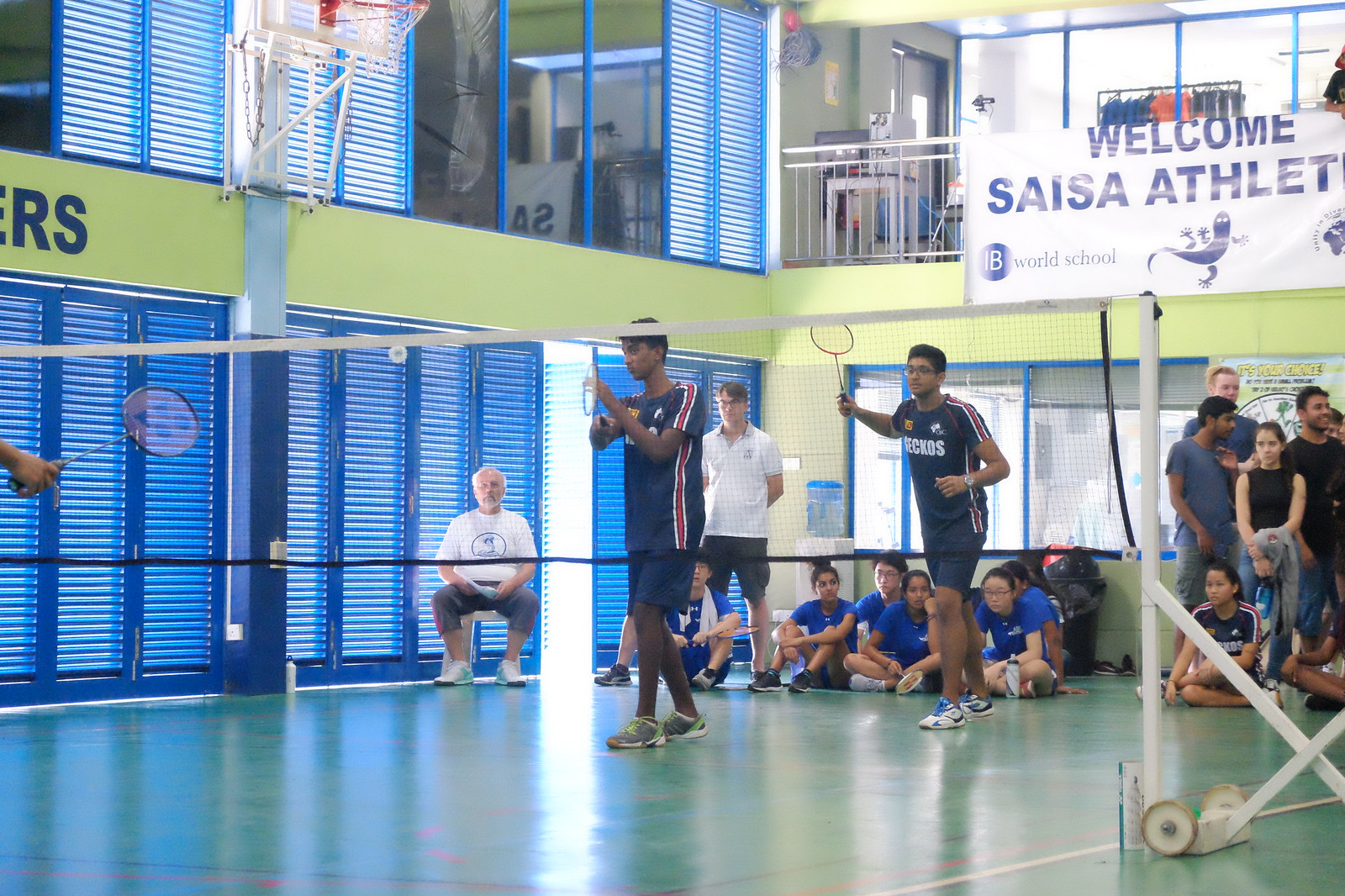The image captures an ongoing doubles badminton match set in a gymnasium with a polished green floor. Central to the scene are two male players of Indian descent, identifiable by their brown skin and black hair, with the player on the right wearing eyeglasses. Both players are dressed in blue uniforms with red pinstripes and the word "GECKOS" emblazoned across their chests. They hold their badminton rackets high in their right hands, poised for action on the right-hand side of the court, backed by a white frame net. 

In the background, a mix of spectators is visible, including several children in lighter blue t-shirts sitting on the ground and an older gentleman in a white shirt seated in a chair. To the left side, the gymnasium features a blue wall with vertical lines and a bordered scalloped design, above which lies a yellow border stretching horizontally. Several windows with blue shades drawn down line the wall, and an additional basketball net can be glimpsed at the top left, indicating the multi-purpose nature of the gymnasium.

In the upper right corner of the image, a prominent blue banner welcomes "SESA Athletes," flanked by sponsor logos. The atmosphere suggests a well-organized sporting event, with every detail from the spectators to the surroundings adding to the live, competitive feel of the scene.